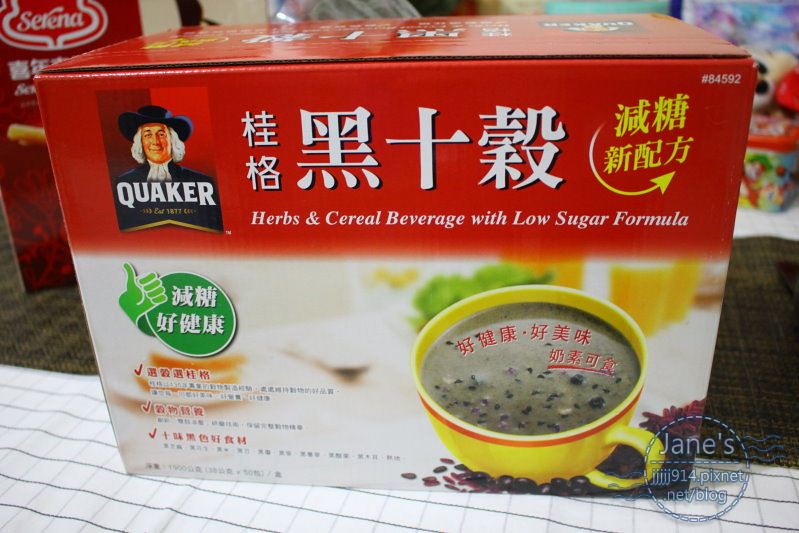The image features a horizontally aligned rectangular picture of a product box on a textured brown fabric background, which seems to be placed on top of a counter or table. In the foreground, there's a white and blue checked towel. To the upper left of the picture, there is a partially visible box labeled "Serena." 

The main focus of the image is a red and white rectangular box of a Quaker product centrally positioned. At the top left corner of the box features the iconic Quaker logo with the Quaker Oats man, including the text "Quaker Established 1877." Directly below the logo, large Asian letters are prominently displayed. Beneath the Asian lettering, the box has the English description "Herbs and Cereal Beverage with Low Sugar Formula."

On the upper right portion of the box, there are more Asian characters in white and yellow colors, including a yellow arrow symbol. Below, a yellow coffee cup with a red rim contains liquid with red Asian writing visible on the surface. Adjacent to this, on the left side, there is a green circle with a thumbs-up symbol and additional Asian characters. More Asian writing in red and black appears below this icon. The background behind the box includes other colorful, though indistinct, items.